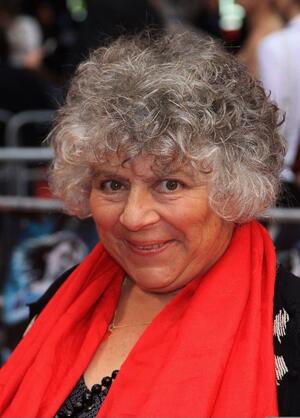This image features an older woman with short, curly hair that has grayed, interspersed with darker shades of black or dark brown. She is smiling warmly, her expression close to a smirk, and her bright demeanor suggests happiness. The woman has brown eyes and tan, yet light skin, indicative of a Caucasian heritage. She is dressed in a stylish black and white top, which is partially concealed by a striking red or possibly orange-red scarf draped around her neck and falling to her front. Additionally, she accessorizes with a beaded black necklace. The portrait cuts off just below her shoulders, focusing closely on her face and upper torso, while the blurry background shows vague outlines of other people and what seems to be a railing. The woman stands out prominently against this less distinct backdrop.